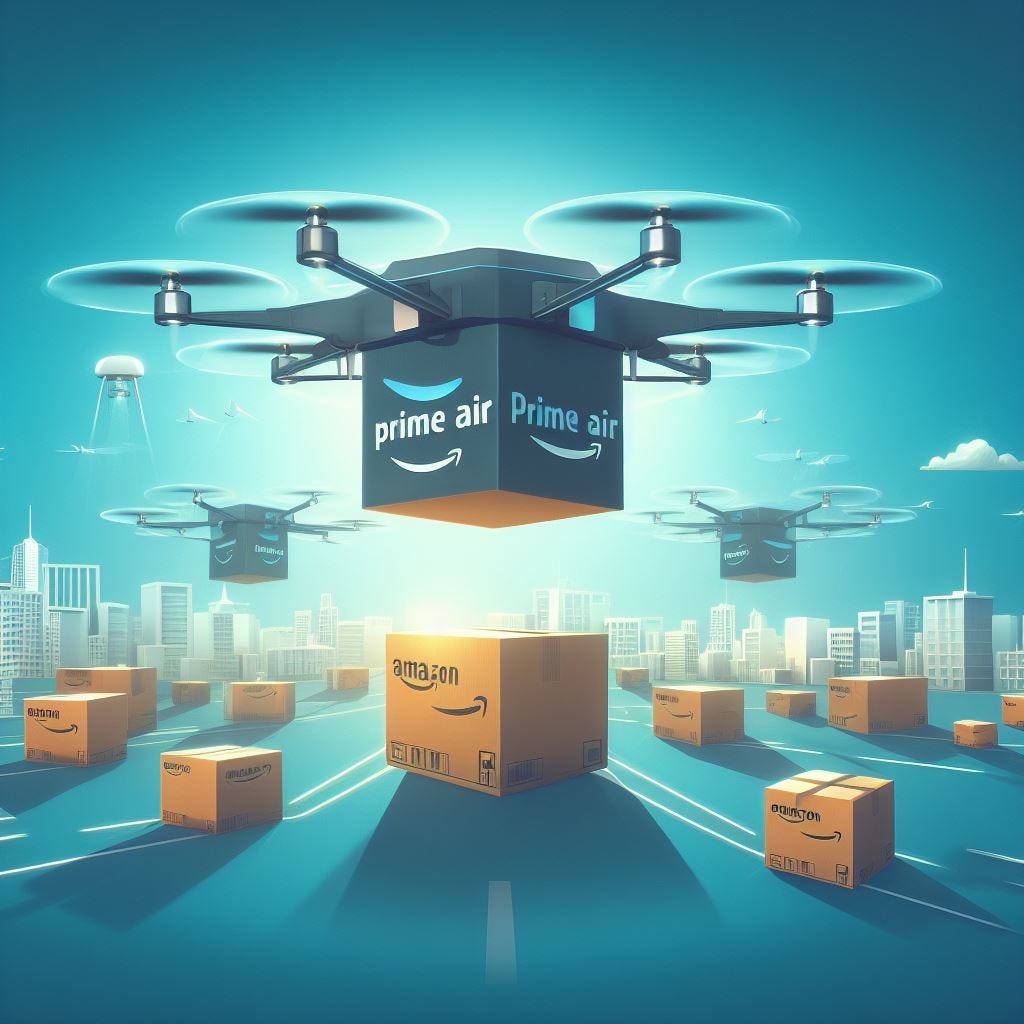The image is a detailed digital illustration, likely a promotional poster for Amazon's Prime Air. It features a futuristic scene showcasing drones delivering packages. The background consists of a gradient blue sky, transitioning from light blue in the middle to darker blue towards the edges. A sprawling cityscape with white and gray skyscrapers, interspersed with blue windows, stretches across the backdrop, with a few clouds adding depth to the scene. 

In the foreground, a blue road marked with white traffic lines is littered with numerous brown Amazon boxes in varying shades, dependent on the lighting and shadows. Each box prominently displays the Amazon logo with its characteristic arrow.

Hovering above the packages are three robotic drones, each equipped with six helicopter-like propellers. The central drone, the largest, bears the Prime Air logo and hovers directly above an Amazon box, suggesting it is mid-delivery or about to pick up the package. Two identical drones can be seen in the immediate background, with seven or eight more scattered farther back. On the far left side of the image, there is a faint outline of a possible aerial deployment center, hinting at the origin of these futuristic delivery drones. The overall blue theme ties the elements together, creating a cohesive and modern aesthetic.